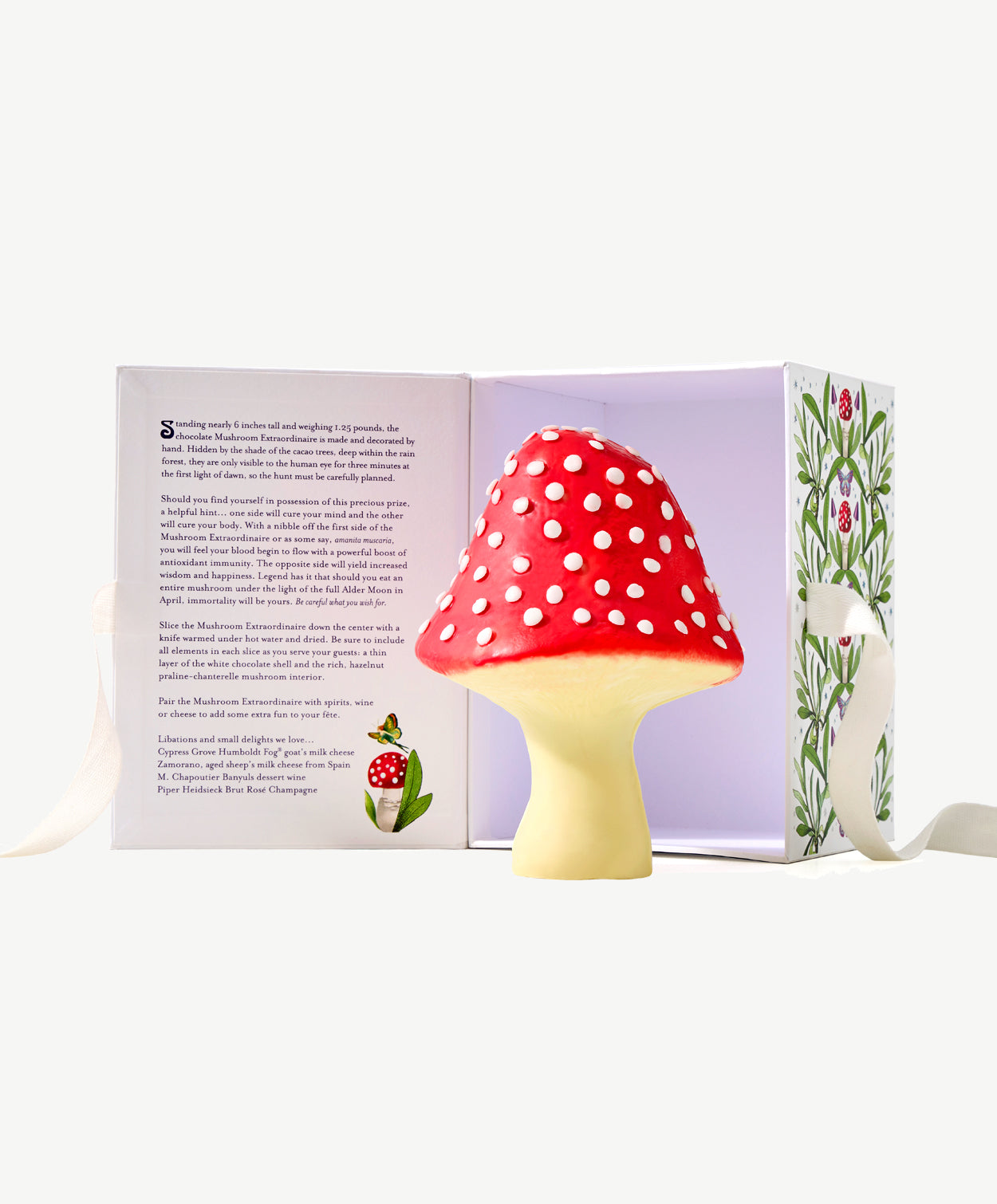The image features an open box with a white background, resembling a shoe box with a hinged flat top. The lid, lined with fabric on either side, reveals a detailed inner cover adorned with extensive text, a butterfly drawing, and a mushroom illustration on the left-hand side. This lid is reminiscent of a book cover when opened. The interior of the box has a light purple hue, contrasting with the decorated exterior showcasing various plants, leaves, and possibly a ladybug. Centrally placed outside this box is a large, artificial mushroom. The mushroom sculpture has a beige stalk and a bright red cap dotted with white polka dots, resembling a whimsical strawberry in form. This decorative mushroom sculpture fits perfectly within the box, suggesting it might be a collectible or a trinket.